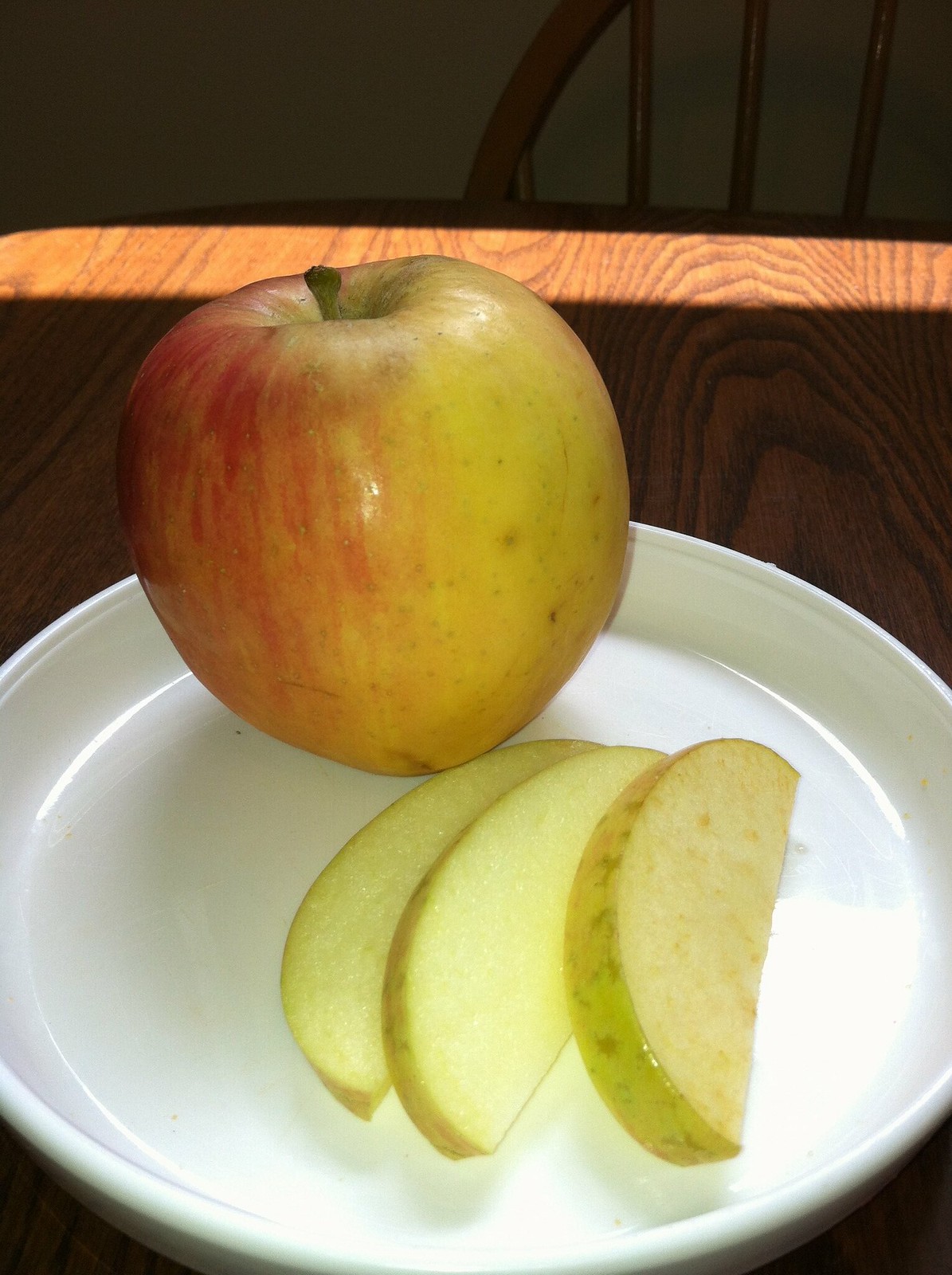A single, uncut apple occupies a white dish placed in the center of the frame, with three neatly sliced pieces of apple arranged in front of it. The background of the image is a wooden table, its intricate grain and rippling patterns clearly visible, traced by where branches once were. A shaft of light illuminates the top of the apple and extends across the table, enhancing the grain's texture. The apple itself is a blend of vibrant colors — predominantly reddish on the left side and transitioning to a bright yellow on the right. The slices, assumed to be cut from the side not visible, display a gradient skin of light green with a hint of pink, while the interior is a crisp white-yellow. The apple's skin shines subtly, indicating freshness. No text distracts from the scene, allowing full focus on the subject. The apple casts a delicate shadow within the dish, which supports the three cut pieces, adding depth to the composition.